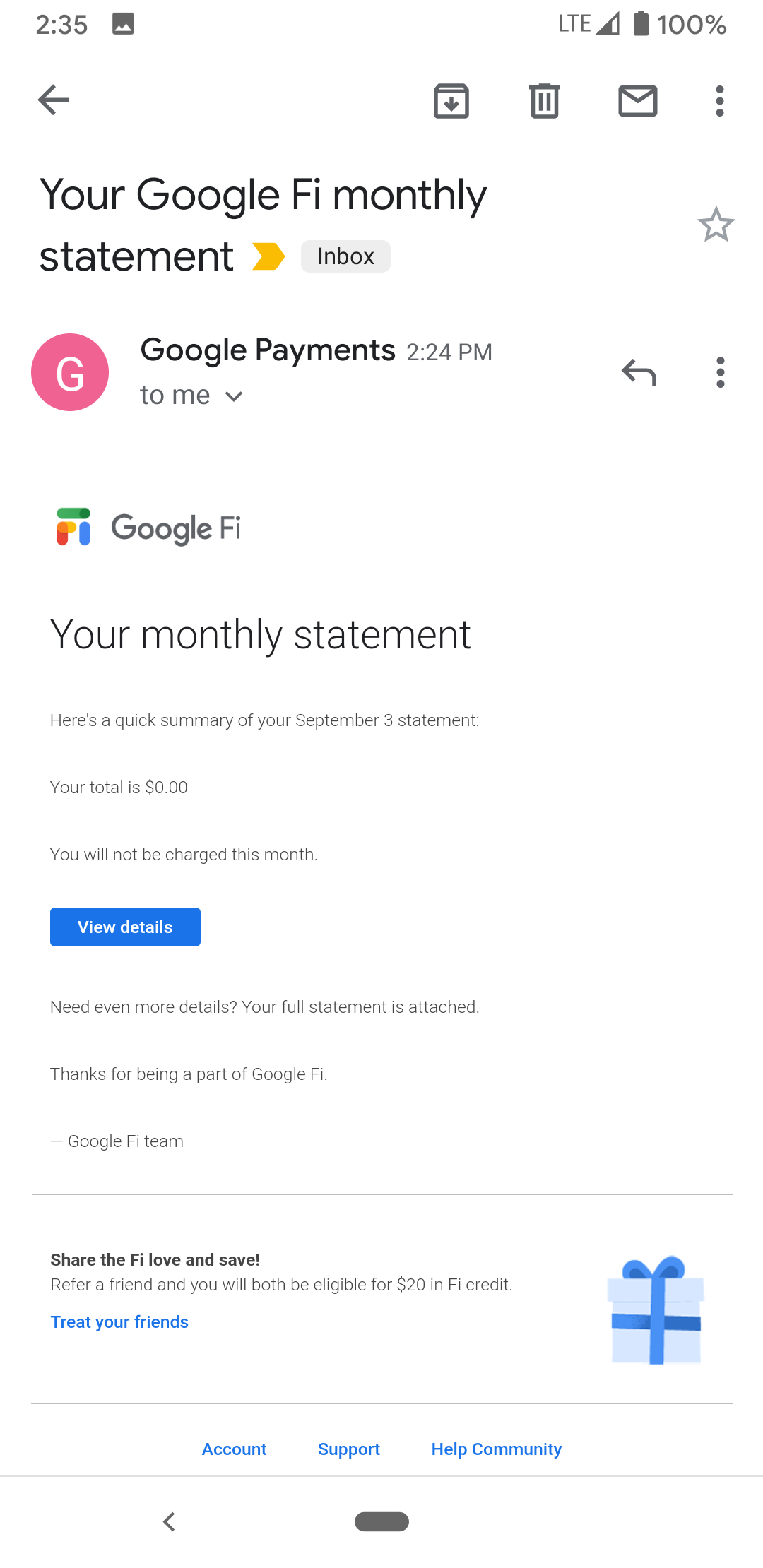The screen displays the heading "Your Google Fi Monthly Statement." Centered below the heading is a purple circle featuring a white "G," which likely represents the Google Payments logo; this logo is also mentioned to the right. The current time is displayed as 2:24 PM. Below the purple circle, there's a colorful Google Fi logo beside a title that reads "Your monthly statement" in smaller text.

The text continues with a brief summary of the statement dated September 3rd, indicating a total of zero dollars, meaning there will be no charges for the month. For those needing more detail, the message notes that a full statement is attached. It concludes with a message of thanks from the Google Fi team. 

The bottom section of the screen includes information about referring friends and the accompanying rewards, accompanied by an unusual logo for friend referrals.